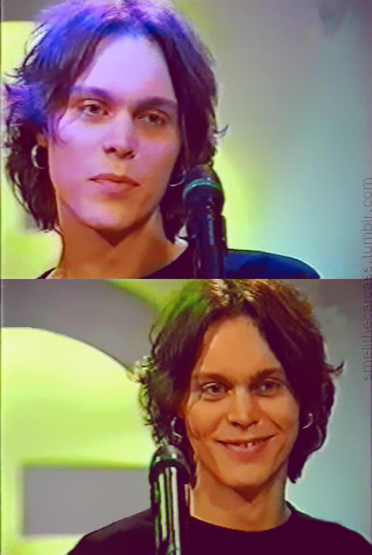The image is a collage divided into two panels, showcasing the same person, identified by their wavy, middle-parted hair, and hoop earrings. In the top panel, the individual appears expressionless, with a microphone positioned to the right of their face. There is a blue light reflecting on their hair, making it appear blue, while their face looks pale white against a blurry, light background with hints of green. They are clad in a black shirt. The bottom panel contrasts this with a smiling expression, revealing their teeth. Here, the hair appears brown with a lime-green light casting a green tint on one side. The background is a blend of grey and green hues, with the person still behind the same black microphone, wearing a brown shirt in this section.